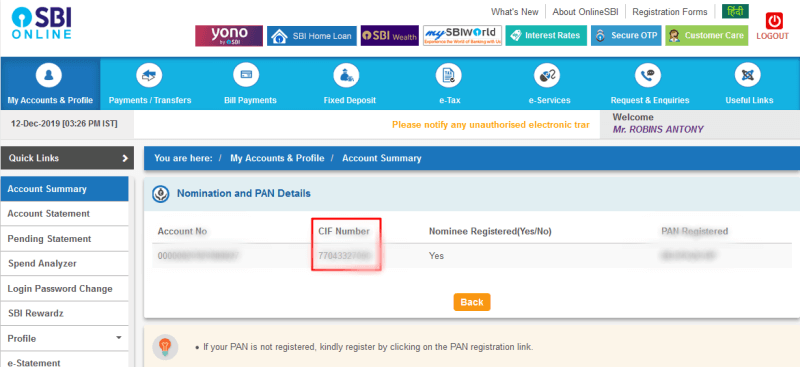**Screenshot of SBI Online Webpage**

The screenshot captures a webpage from SBI Online. On the top left corner, there is a logo featuring a blue circle with a white dot and a line descending in the shape of an upside-down 'C'. Next to the logo, moving rightward, is "SBI Online" followed by the word "YONO" inside a reddish-purple box. Adjacent to this is a blue box with a house icon and the label "SBI Home Loan". Further right is a purple box labeled "SBI Wealth", succeeded by a white box with the text "My SBI Wealth". Continuing in this sequence is a teal box labeled "Interest Rates", next to which is a blue box titled "Secure OTP", followed by a green box for "Customer Care". At the far right, a red power button marked "Logout" is visible.

Directly below this row, there is a blue navigation bar with tabs titled: "My Account," "Profile," "Payment Transfers," "Bill Payments," "Fixed Deposit," "E-Tax," "E-Service," "Inquiries," and "Useful Links". Below this bar, the date and time display reads "December 12, 2019, 3:26 PM IST". Text beneath this advises notifying any unauthorized electronic transactions. To the right of this advisory, a personalized message reads "Welcome Mr. Robbins Anthony".

On the left side below this message, a quick links section lists: "Account Summary," "Account Statement," "Pending Statement," "Spending Allowance," "Logged-in Password Change," "SBI Rewards Profile," and "E-Statement". To the right, a blue box indicates "You are here: My Account Profile - Account Summary". Below this, a lighter blue box contains details for "Nomination and PAN Details," listing: Account Number (blurred), CIF Number (blurred), Nominee Registered (Yes), and PAN Registered (blurred). The CIF number is highlighted by a red box. There is also an orange "Back" button in this section with a note: "If your PAN is not registered, you can register by clicking on the PAN registration link".